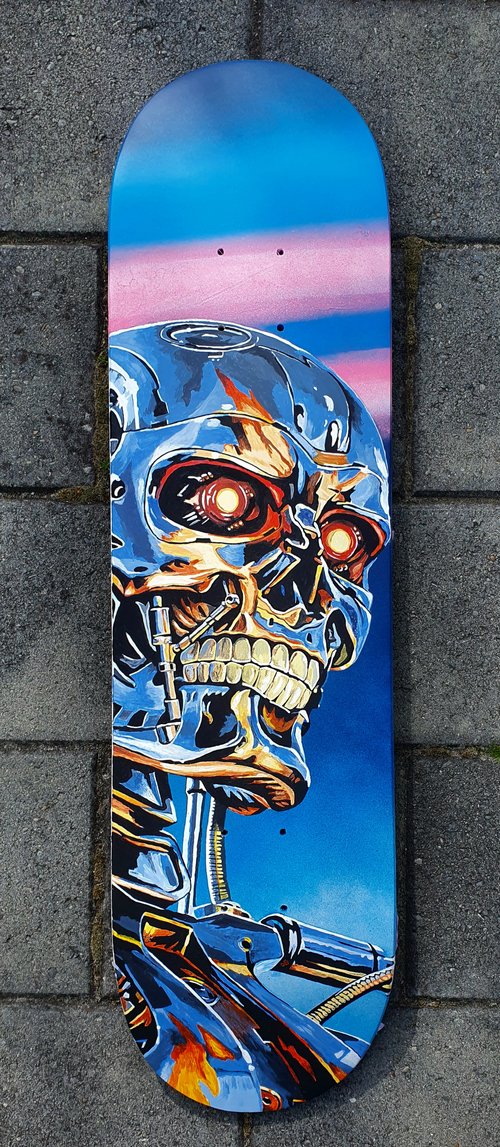The image features a skateboard without wheels, resting on a gray block pavement with black mortar in the seams. The board has a neon blue background, adorned with neon pink stripes. Dominating the deck is an intricate depiction of a metallic skeleton or android, reminiscent of the Terminator exoskeleton. The android has a skull-shaped head with exposed, human-like white teeth, and piercing red eyes with white centers, giving it a strikingly serious and somewhat frightening appearance. The robotic figure includes additional mechanical details such as a pneumatic line connecting its jaws, various cables, and hydraulic fixtures around its neck and shoulders. The upper part of the torso is visible, showing a complex array of shades of blue, hinting at its artificial and robotic nature. The contrasting pink lines in the background enhance the futuristic and eerie visual of the skateboard design.